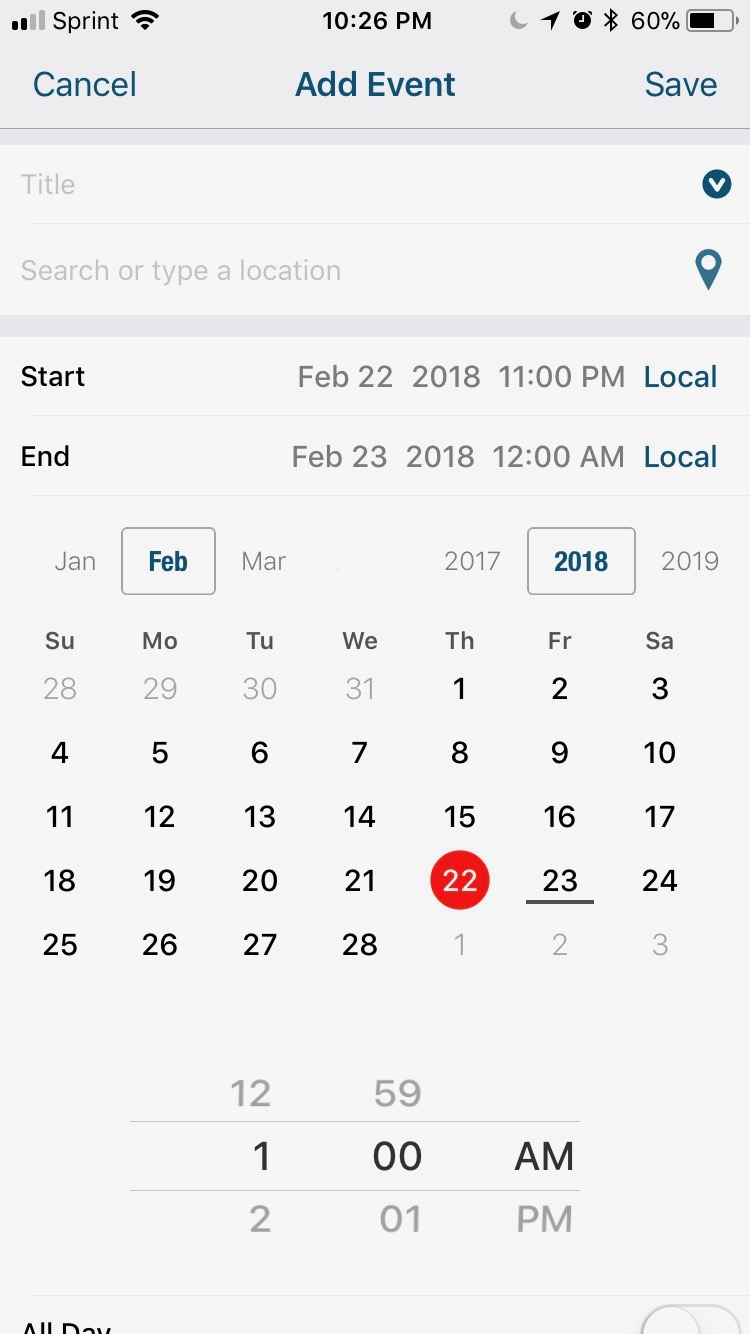This is a detailed screenshot of a calendar event creation screen on a mobile device. 

At the top of the screen, there's a gray status bar displaying "Sprint" along with a Wi-Fi symbol, two signal strength bars, the time "10:26 p.m.", and a series of icons including a crescent moon, an airplane, an alarm clock, and a Bluetooth symbol. The battery indicator shows 60%.

Below the status bar, there's a blue strip with the options "Cancel," "Add Event," and "Save."

Moving down, two gray input fields are separated by a thin gray line. The first field, labeled "Title," features a blue and white circle icon, while the second field, labeled "Search or type a location," has a blue location pin icon.

Further down, we see event timing details. In black text, it states "Start: February 22, 2018, 11 p.m. Local" and "End: February 23, 2018, 12 a.m. Local," with "Local" highlighted in blue.

Next, there is a date selector highlighting February 2018. "Jan," "Feb," and "Mar" are options available, with "Feb" highlighted in blue. The years "2017," "2018," and "2019" are shown, with "2018" highlighted.

The calendar grid below shows the last few days of the previous month in light gray, and the current month’s days in black text. The date "22" is circled in red with white font.

Lastly, there is an alarm setting for "1 a.m." and a gray toggle button labeled "All day," with the toggle currently set to off.